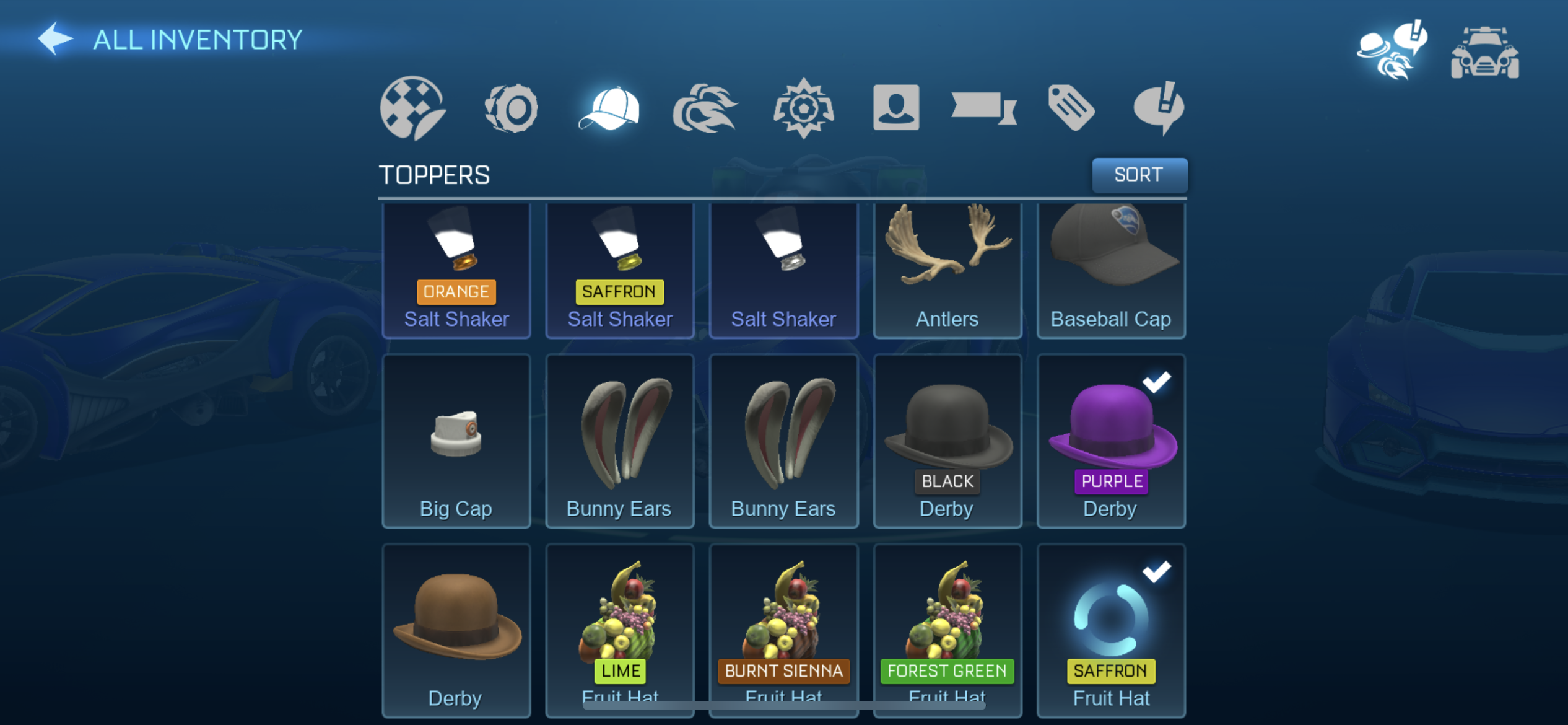The image is a color screenshot from what appears to be a mobile racing video game, showcasing an inventory screen dedicated to customizable headwear for an avatar or character. The interface is primarily overlaid on a dark blue background, with slight visibility of cars in the background, hinting at a racing game context. The screen prominently displays various headwear items under the category "Toppers," with numerous hats listed, including Black Derby Hat, Bunny Ears, Antlers, along with colorful items described as Orange Salt Shaker, Saffron Salt Shaker, and more. 

At the top left corner, there's a label "All Inventory" accompanied by a white arrow pointing to the left, indicating navigation options within the inventory. The top right corner features two icons, though their purpose is unclear. Some headwear items, such as the Purple Derby and Saffron Fruit Hat, are marked with white check marks, possibly indicating they are currently selected or equipped. Other tabs in the menu suggest additional customization options, like tires and speed, further supporting that this is a racing game inventory screen.